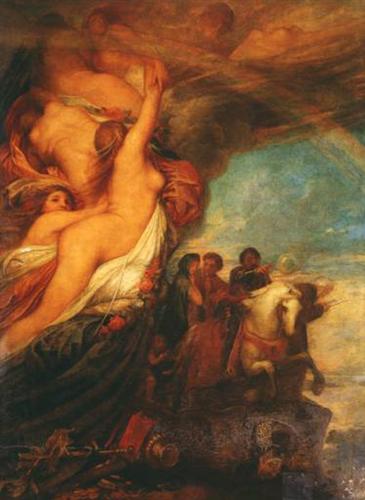The image depicts a Renaissance-style painting characterized by muted yet colorful tones. On the left side, a prominent column of naked human bodies, dominated by a nude woman in a side profile stretching upwards, forms a whirlwind-like ascension into the sky. This woman, with long reddish-brown hair cascading down her back, holds a white blanket that drapes around her body, and is closely trailed by a child, also gripping a white blanket and floating behind her. The column blends into a cloud of bodies and whitish smoke, ascending higher into a blue sky dotted with clouds. On the right side, several indistinct figures dressed in Renaissance-era clothing ride white horses adorned in elaborate gear, suggesting nobility. The painting, slightly yellowed and blurry with age, features a desert-like setting under a clear blue sky with a subtle rainbow in the background. The composition suggests a biblical or otherworldly scene, blending earthly and celestial elements.